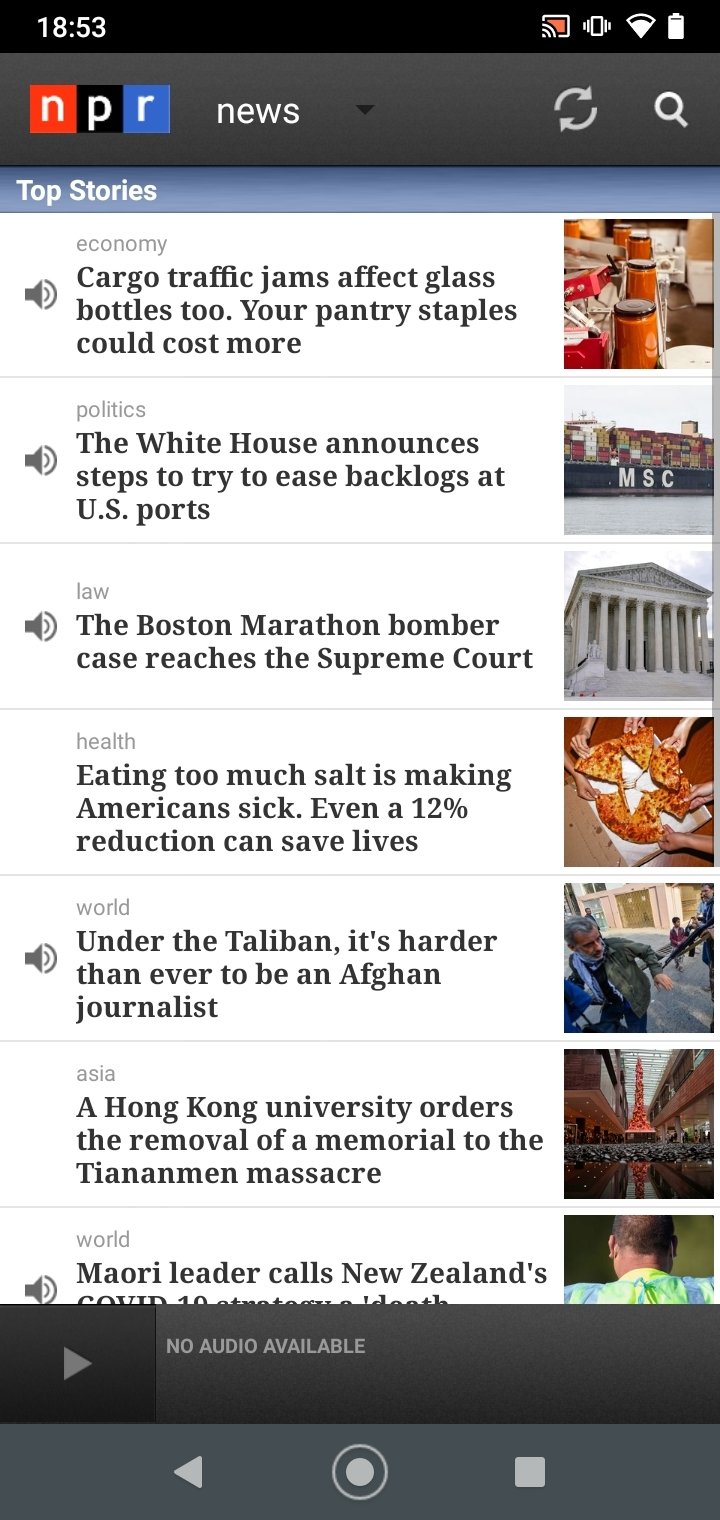This image displays the screen of a smartphone showcasing a website with a full battery charge and a strong connection signal. The time displayed on the phone is 18:53. The website is identified as NPR News, featuring several headlines across different sections. 

In a vivid outline, the interface comprises a red box bordered in gray with curved lines at its lower part. Although its function remains unclear, the primary focus is on the news content.

Under the "Top Stories" section, the headlines read:

- **Economy**: "Cargo traffic jams affect glass bottles too. Your pantry staples could cost more."
- **Politics**: "The White House announces steps to try to ease backlogs at U.S. ports."
- **Law**: "The Boston Marathon bomber case reaches the Supreme Court."
- **Health**: "Eating too much salt is making Americans sick. Even a 12% reduction can save lives."
- **World**: "Under the Taliban, it's harder than ever to be an Afghan journalist."
- **Asia**: "A Hong Kong University orders the removal of a memorial to the Tiananmen Massacre."
- **World**: "Maori leader calls New Zealand's COVID-19..." (with the remainder of the headline cut off).

Towards the bottom of the screen, there is a gray box indicating "No audio available." Below this is another gray box featuring the usual navigation icons commonly found on smartphones.